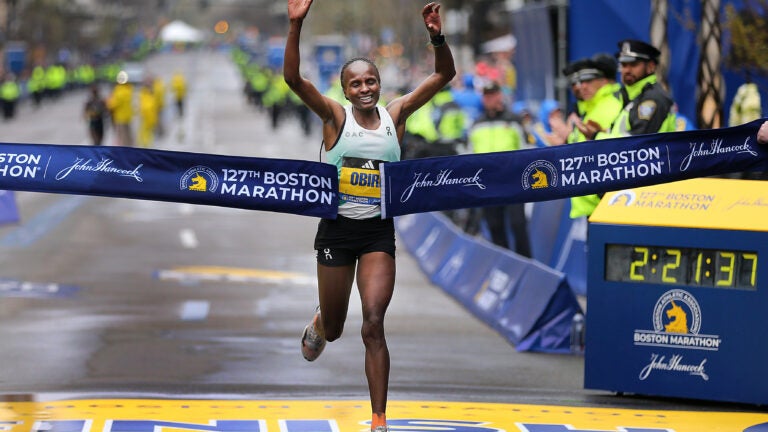The image captures a triumphant moment at the 127th Boston Marathon with an African-American woman in her 60s or 70s crossing the finish line. She has dark brown skin, is dressed in a white tank top, short black shorts, and orange sneakers. She's breaking through a blue ribbon adorned with the John Hancock logo and a golden unicorn emblem, accompanied by the event's title, "127th Boston Marathon," in white text. The woman exudes immense emotion, with her hands raised, eyes closed, and mouth open, possibly shedding tears of joy as she achieves victory. She sports a yellow sticker with "OBIR" on her outfit. To her right, an LED timer on a blue box with a yellow roof displays "2:21:37" and the Boston Marathon logo. Behind her, blurred runners indicate her winning status. Police officers in reflective yellow and neon vests maintain security, amidst the rainy backdrop, with barriers ensuring crowd control. The ground beneath is marked with "FINISH" in blue letters with a white outline, completing the scene of this monumental and emotional victory.